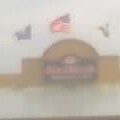The image is a small, fuzzy depiction of a tented structure with distinctive architectural elements. At the center of the structure is a rounded section resembling a cupola, crowned by a prominent red flag fluttering at the top. Flanking the central cupola are two flat-topped wings. In front of the structure, there appears to be a shorter element, possibly a fence. Two additional smaller flags are visible on either side of the cupola: one is bluish, and the other, triangular in shape, has an indeterminate color due to the angle and quality of the image. The specific nature and purpose of the structure remain unclear.